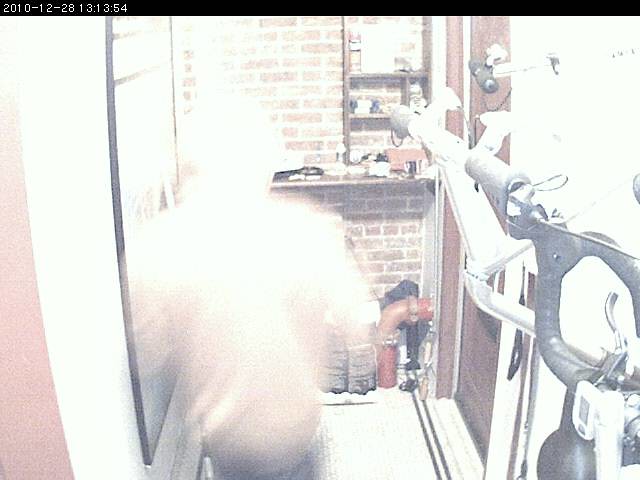This surveillance camera screenshot, dated "2010-12-28 13:13:54," features an overexposed and washed-out image, making it difficult to discern details. The scene appears to depict an individual entering a garage or front door area. A figure wearing a light-colored shirt can be seen walking away from the camera, though their appearance is blurry. The floor and sides of the area are cluttered with various metal tools and supplies. On the right side of the image, a brown door is visible, while a brick wall is situated straight ahead.